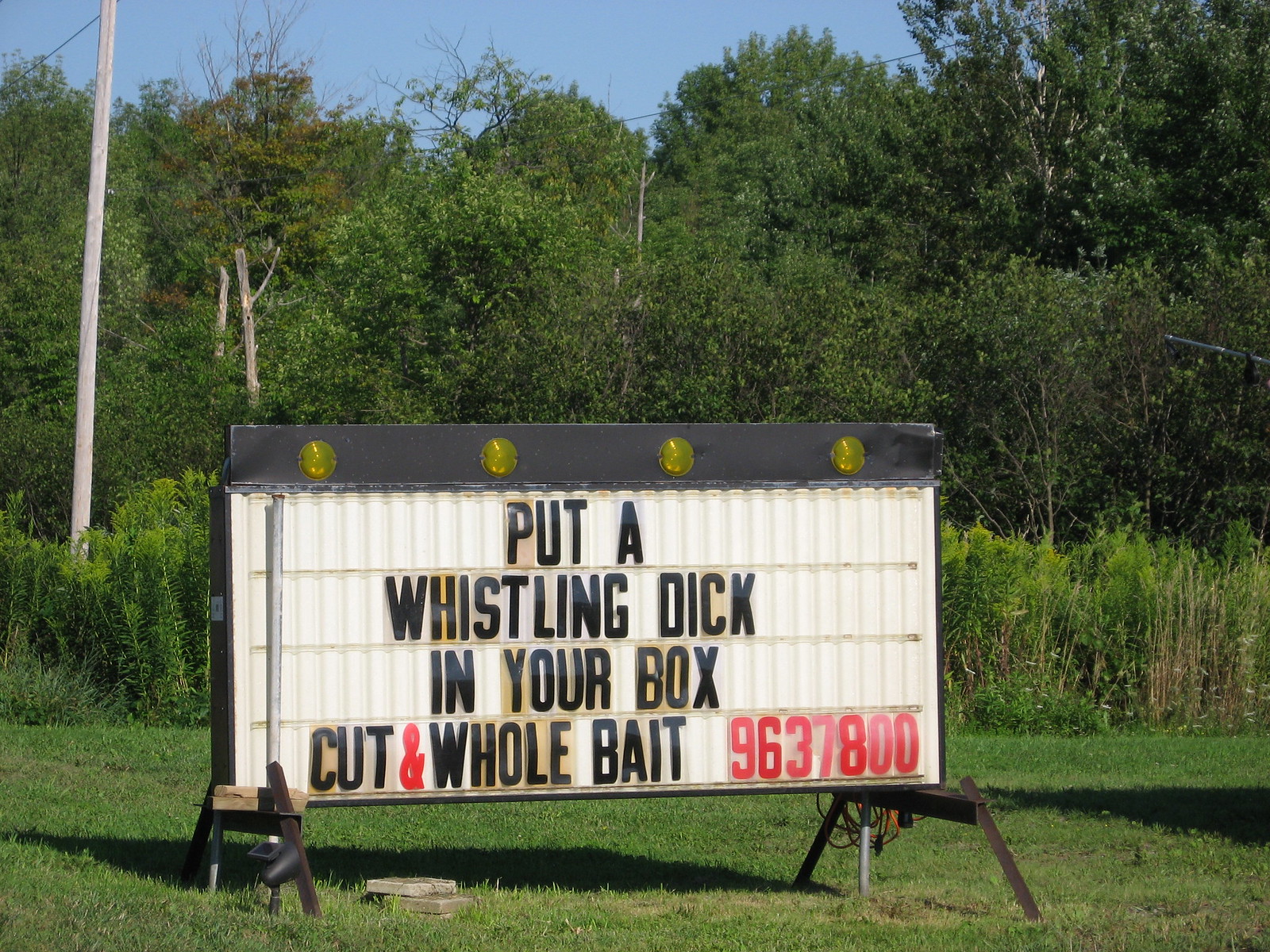This daytime photograph features a unique sign balanced on two black metal framework supports. The sign has a white background with a black top border and includes four round lights, which are unlit due to the daylight. The text on the sign, written with interchangeable black and red letters, reads: "Put a Whistling Dick in Your Box. Cut and Whole Bait. Phone Number 963-7800." The sign is positioned on a grassy lawn that leads to a dense woodland area with lush, dark green foliage. In the upper left corner of the image, a solitary gray telephone pole is visible against the backdrop of trees.